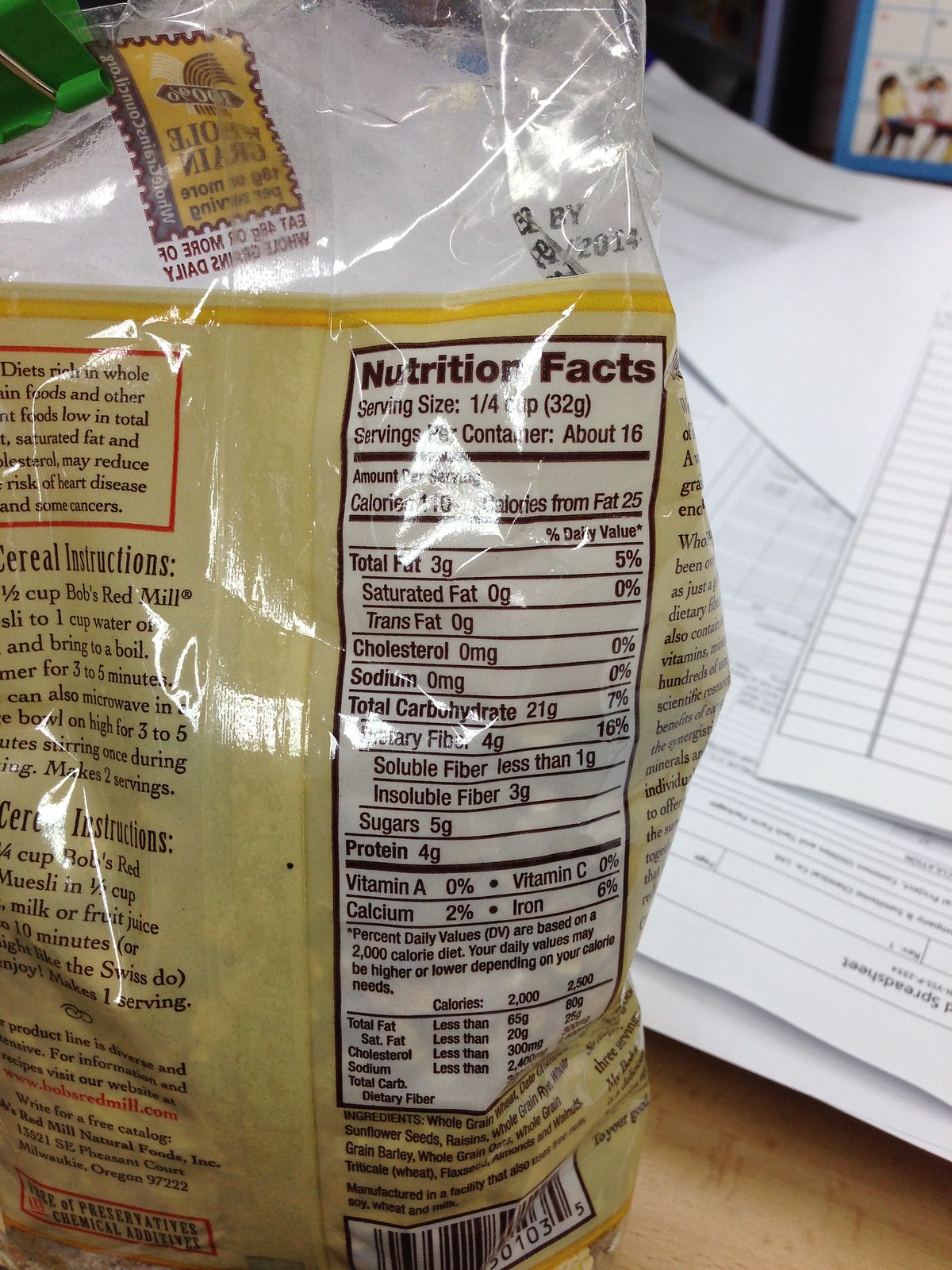This is a detailed photograph of the back of a package of Bob's Red Mill Muesli. The package, made of transparent plastic, is filled with the muesli and features a greenish-gold color design on the lower half. A prominent white panel highlights the nutrition facts, detailing that the serving size is 1/4 cup (32 grams) and there are approximately 16 servings per container. The panel indicates that each serving contains 3 grams of total fat, 0 milligrams of cholesterol, 0 milligrams of sodium, 21 grams of carbohydrates, 4 grams of dietary fiber (including less than 1 gram of soluble fiber and 3 grams of insoluble fiber), 5 grams of sugar, and 4 grams of protein, with no Vitamin A or C, 2% calcium, and 6% iron. Despite some light glare making parts of the package harder to read, the details are clearly outlined. Below the nutrition facts, the ingredients are printed in small letters, and a barcode is situated at the bottom. On the left side of the bag, instructions for preparing the cereal, a brief history of Bob's Red Mill, and the benefits of eating such wholesome foods are included. The packaging rests on a brown table, with some white documents faintly visible in the background and an expiry date noted at the top of the image. The bottom section also features an orange border, adding a finishing touch to the detailed packaging.